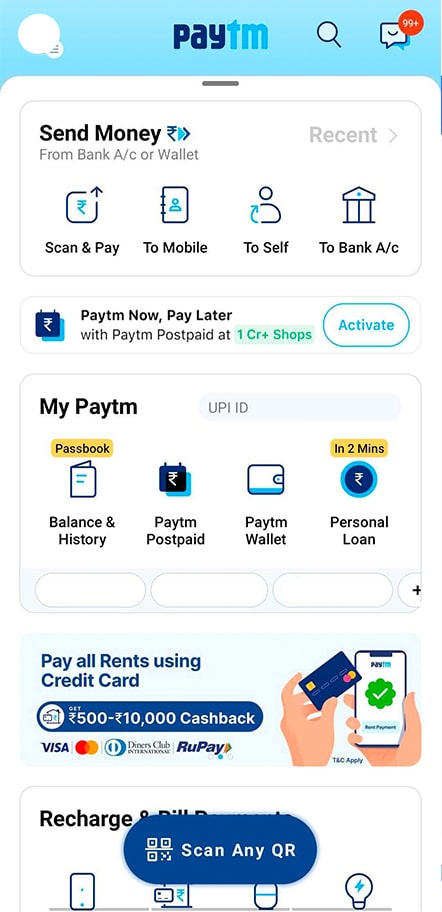The image starts with a light blue header that contains a white circle intersected by a smaller segment at the bottom, followed by the text "PayTM". To the right, there is a magnifying glass icon representing search, and a squarish cat icon with a red circle indicating "99+" notifications.

Below the header, there is a section titled "Send money from Bank A/C or Wallet". This section includes the word "Recent" followed by an arrow pointing to the right. Beneath this text, there are four icons with accompanying labels: "Scan & Pay," "To Mobile," "To Self," and "To Bank A/C".

The subsequent section promotes "PayTM PostPaid," stating "PayTM Now, Pay Later with PayTM PostPaid at 1 CR+ Shops," accompanied by a curved rectangular button labeled "Activate".

Further down, there is a section titled "My PayTM" which includes a text box with the placeholder "UPI ID" in gray text. Following this are several icons with their respective labels: "Balance & History," "PayTM PostPaid," "PayTM Wallet," and "Personal Loan".

The next section prompts users to "Pay All Rents Using Credit Card" with a cashback offer ranging from "500 to 10,000" in the specified currency. This section features an illustration of a person holding a phone in their right hand and a credit card in their left hand. The phone screen displays a circular green area with a white checkmark.

At the very bottom, a partially visible section seems to involve recharges, but is obscured by a blue rectangular button that reads "Scan Any QR".